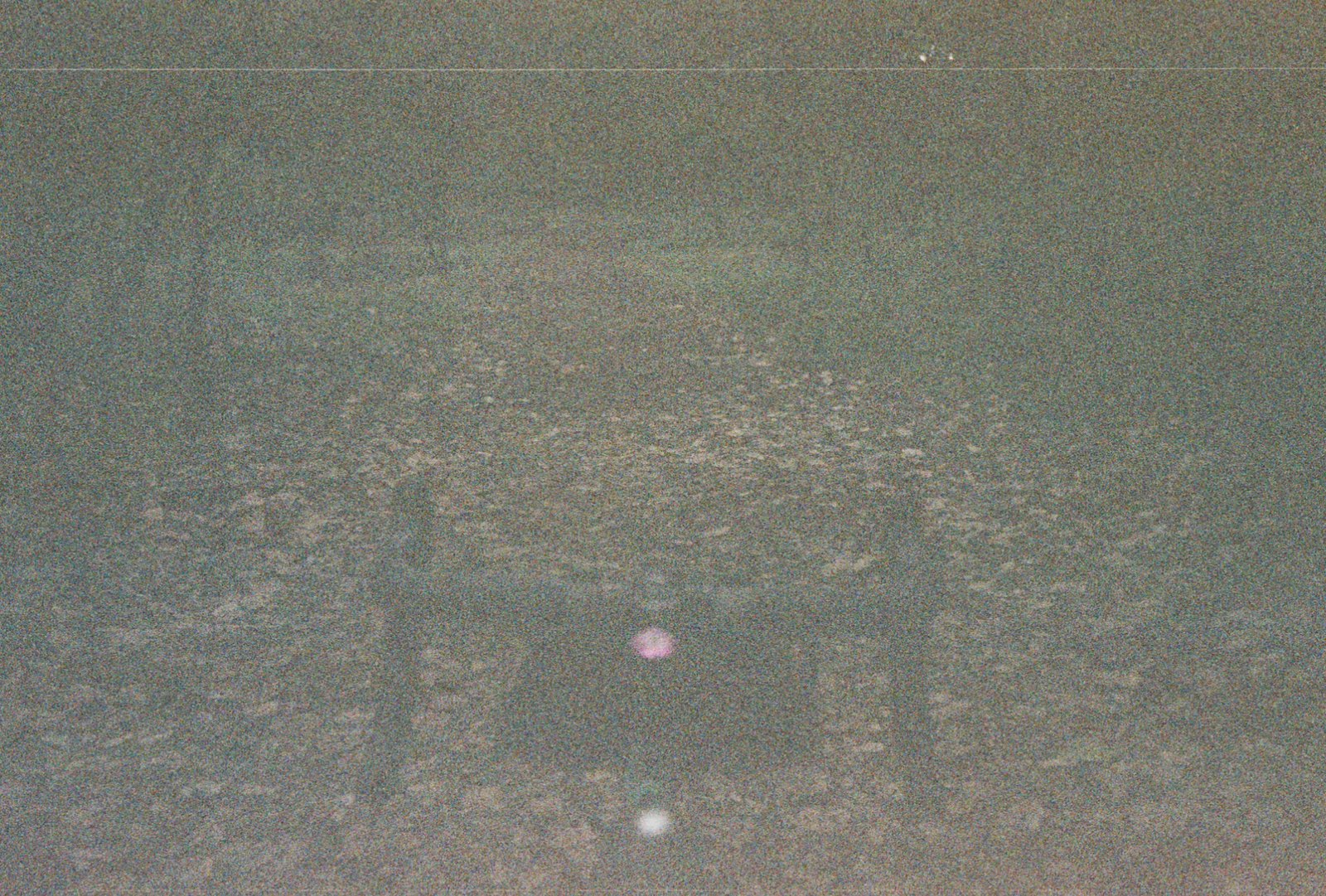In this extremely hazy image, a mystical shrine-like structure is barely discernible in the foreground. Two vertical stakes emerge from the ground, connected by a horizontal bar, resembling an altar. Just underneath the center of this bar, a vague pink detail can be observed, possibly a decorative element. Below this, a darker, indistinct object contrasts with the murky surroundings. Further down, a soft white light emanates, casting a mysterious glow on the area below. The ground is strewn with brown leaves, suggesting a leaf-covered pathway, likely a dirt path winding through a wooded area. The entire scene is enveloped in a greenish fog, particularly thick around the pathway, adding an ethereal quality to the already enigmatic image.